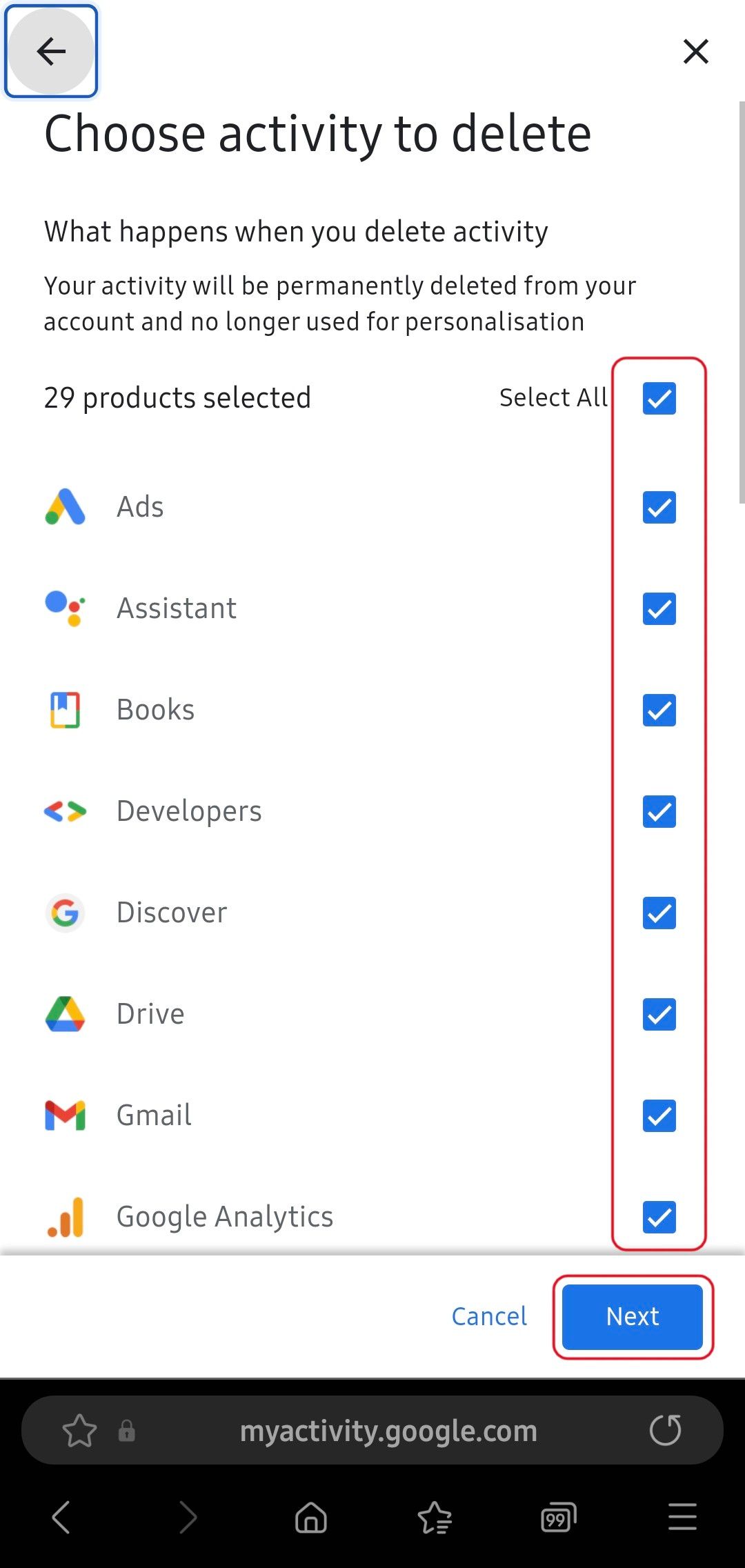This image is a screenshot from the My Activity section of a Google account, captured on a mobile device. At the top of the screen, there is an option labeled "Choose activity to delete." Below this, a message states: "What happens when you delete activity? Your activity will be permanently deleted from your account and no longer used for personalization." The user has selected 29 products to delete, as indicated by the text "29 products selected" and a "Select all" option, with blue check marks next to each product on the right side. 

The left sidebar lists various Google services, including Ads, Assistant, Books, Developers, Discover, Drive, Gmail, and Google Analytics. On the right side of the screen, buttons for "Cancel" and "Next" are present, guiding the user through the deletion process. At the very bottom, the URL "myactivity.google.com" is displayed along with a small star icon. 

The bottom navigation bar features different icons including arrows, a house, a star, a figure resembling a cassette tape, and a menu icon with three lines. The blue check marks next to every listed product indicate that the user has chosen to delete all of their activities across these services. This screenshot is essentially about managing and deleting user activity from their Google account.